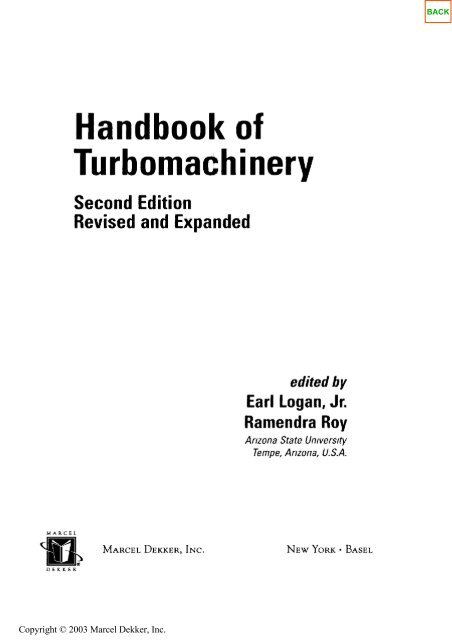The image is the cover of a textbook entitled "Handbook of Turbo Machinery." It prominently features black text against a white background. At the top, the title "Handbook of Turbo Machinery" is printed in black, followed by "Second Edition" and "Revised and Expanded." The lower right portion of the cover lists the editors: "Edited by Earl Logan, Jr.," and "Ramendra Roy," along with their affiliation, "Arizona State University, Tempe, Arizona, USA." Further down, the publisher's name, "Marcel Decker Incorporated," is noted with locations "New York" and "Basel." Additionally, a detail indicating "Copyright 2003, Marcel Decker Incorporated" is present. There's an element on the top right corner marked with green letters and a red square.